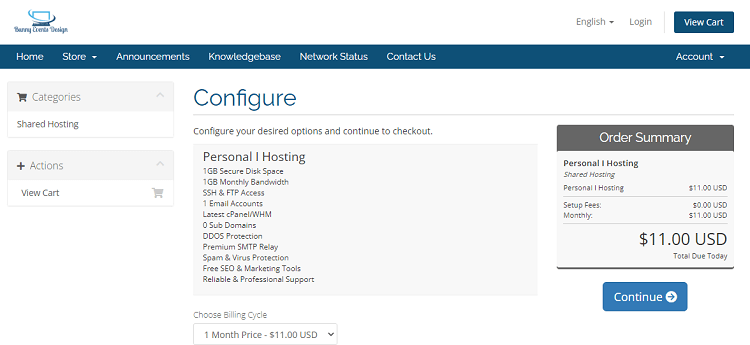The image displays a website interface for a company offering computer hosting services. In the upper left corner, there's a small logo depicting a coffee cup and a computer, possibly indicating the company's name, which appears partially clarified as "Sunny Gara." Below the logo, the site features navigational links for Home, Store, Announcements, Knowledge Base, Network Status, and Contact Us.

The page depicted is an Order Summary for personal hosting services. The summary indicates that the customer has selected a hosting plan priced at $11 per month, with no setup fees. The total amount due today is $11. A prominent blue button marked "Continue" is situated below the order details.

In the main body of the page, there is an instruction that reads, "Configure your desired options and continue checkout." The personal hosting plan includes 1 GB of secure disk space, 1 GB of monthly bandwidth, SSH and FTP access, and 1 email account. The screenshot suggests that the person is in the process of purchasing these hosting services from the company.